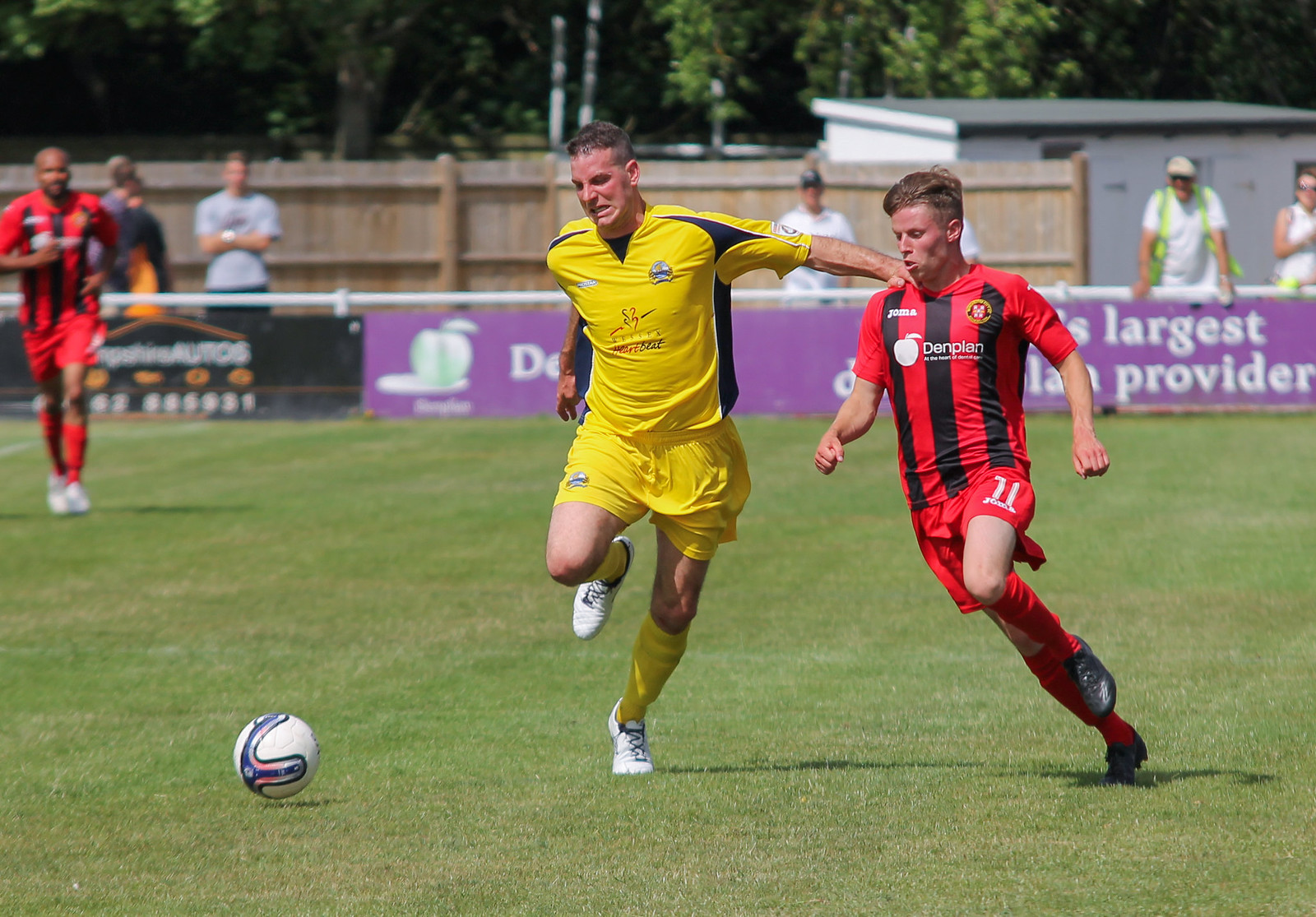The image captures a dynamic moment on a green soccer field during a sunny day, where two players are intensely vying for a white soccer ball with blue details. The player on the left is donning a complete yellow uniform accented with blue details, yellow socks, and white shoes. His expression is focused and determined, with his right arm outstretched, grabbing the shoulder of the opposing player to impede his progress. This opposing player is outfitted in a red and black striped jersey with "DenPlan" written across the chest, red shorts, red socks, and black shoes. In the backdrop, another player from the red and black team can be seen jogging, possibly playing defense. The field is lined with various advertising boards – a standout being a purple sign with white text and a black sign symbolizing an auto company. Spectators are standing behind these signs, indicating there might not be seating on this side of the field. Additionally, a building and foliage are visible behind the fence enclosing the spectators.